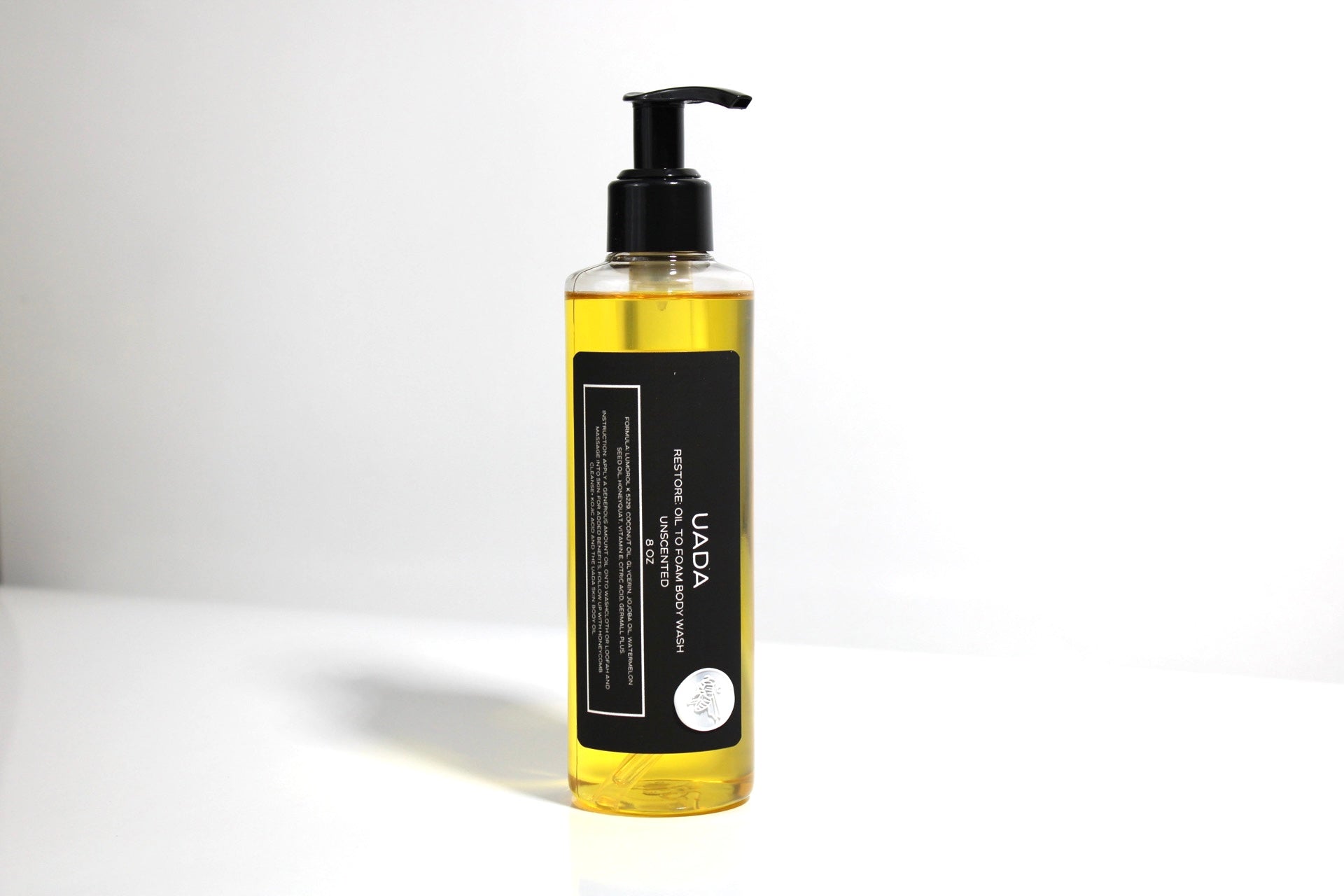The image depicts a clear plastic cylindrical pump bottle filled with a gold-colored liquid, likely a soap or body wash. The bottle, standing upright on a white counter against a white wall, features a black lid with a cylindrical pump top. A vertical black label runs down the front, displaying the text "UADA" in all capital letters, with further smaller text indicating it is a "restore oil to foam body wash, unscented, eight ounces." The backdrop is completely white, giving the image a clean, minimalist aesthetic, and a slight shadow is cast to the left of the bottle, enhancing its three-dimensional appearance.